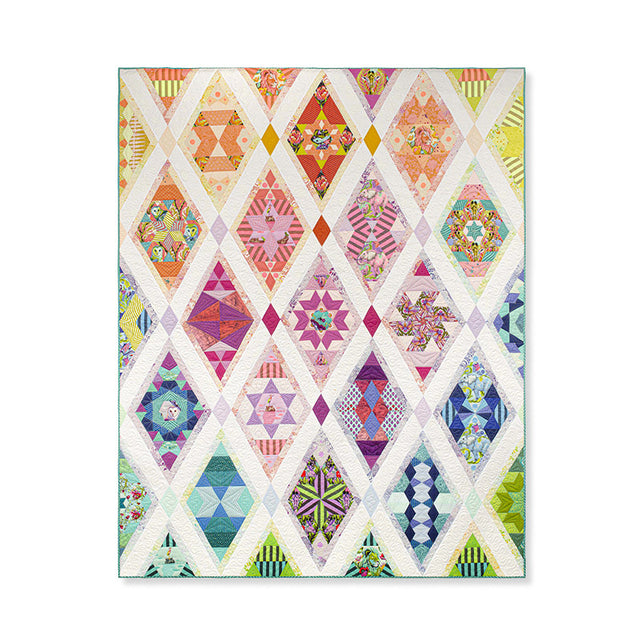This vibrant quilt showcases an intricate and colorful design. The background features an array of white diamond shapes, each containing a unique color and pattern. Central to the design is a striking motif: a red background holding a gold star, with a blue center. Interspersed throughout the quilt are various hues, including bold purples, soft yellows, deep blues, and a myriad of others like pink, orange, and green. The patterns are equally diverse, with floral elements adding a specific charm. Each diamond's distinct combination of colors and designs makes the quilt an eye-catching piece that radiates warmth and creativity.